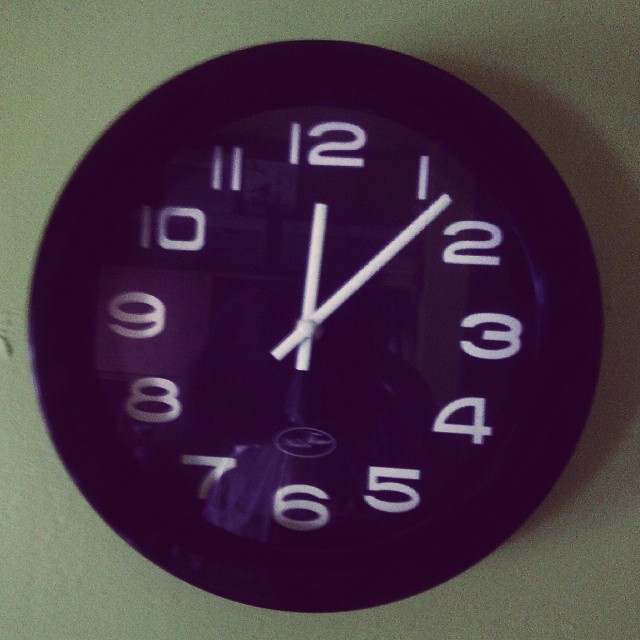A modern wall clock stands out prominently on a gray wall. The clock face is designed to resemble a royal purple plate, accented by a darker rim around its edge. White, Arabic numerals clearly indicate the time, which reads 12:06. Above the numeral six, there is a logo of the clock's maker, although it is blurred and difficult to decipher. The overall composition includes the clock casting a soft shadow onto the wall. The plastic covering of the clock reflects the image of someone taking a photograph, making it slightly challenging to discern precise details. However, in the reflective background, one can identify modern white bookcases equipped with sleek white cabinets and baskets for organizational purposes.